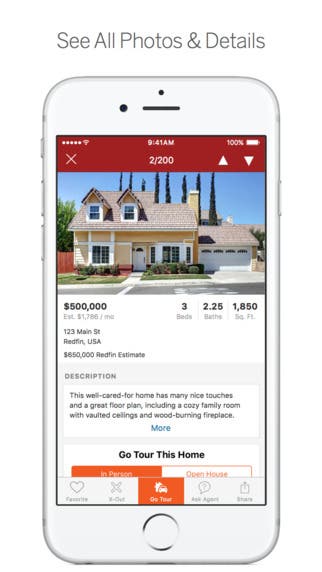This image is a detailed screenshot of a real estate listing displayed on an older model white iPhone, possibly an iPhone 7. The screenshot has a white background with gray text at the top that reads "See all photos and details."

At the top of the screen, there is a dark red banner with a white "X" icon for closing. This banner indicates that the image shown is "2 of 200," and has white arrows pointing upward and downward for navigation.

Below the banner, a picture of a single-family home with a lawn is featured, suggesting that the focus of the listing is on this property. The listing price is prominently displayed as $500,000. Further details about the home include three bedrooms, 2.25 bathrooms, and a total area of 1,850 square feet. The property address appears to be 123 Main Street, Redfin, USA, and the Redfin estimate stands at $650.

Further down, within a gray box labeled "DESCRIPTION," the text describes the home as well-cared-for, highlighting its cozy family room with vaulted ceilings and a wood-burning fireplace. Below this description, blue text saying "More" invites users to read further.

Additional call-to-action buttons include a white box encouraging users to "Go tour this home," and an orange button with white text labeled "In person." Another clickable option is an orange text on a white background, advertising an "Open House."

At the bottom of the screen, there are various menu icons that likely represent different functions. These include a heart, an "X," a car, a question bubble, and a share button, offering interactive options for users to save, reject, find directions, ask questions, or share the listing respectively.